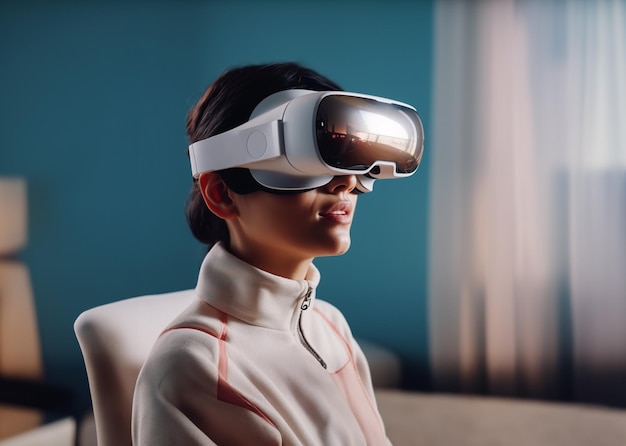In the photograph, a woman with dark, low-bun hair and medium-light skin is immersed in a VR experience, wearing what appears to be an Apple-brand VR headset. She dons a white athletic jacket with light peachy-orange detailing and a zippered front, giving it a fleece-like thermal quality. The close-up shot captures her upper body as she sits on a white, modernistic-looking chair. Her head is turned slightly to the right, and her expression is neutral, suggesting a focused engagement rather than emotional response. The VR headset has a glossy, glass front, reflecting bluish and orangey hues, indicating the surrounding environment. Behind her, the background is softly blurred, featuring a light blue wall, shadows, and partially transparent white curtains, which enhance the serene and modern atmosphere of the room.